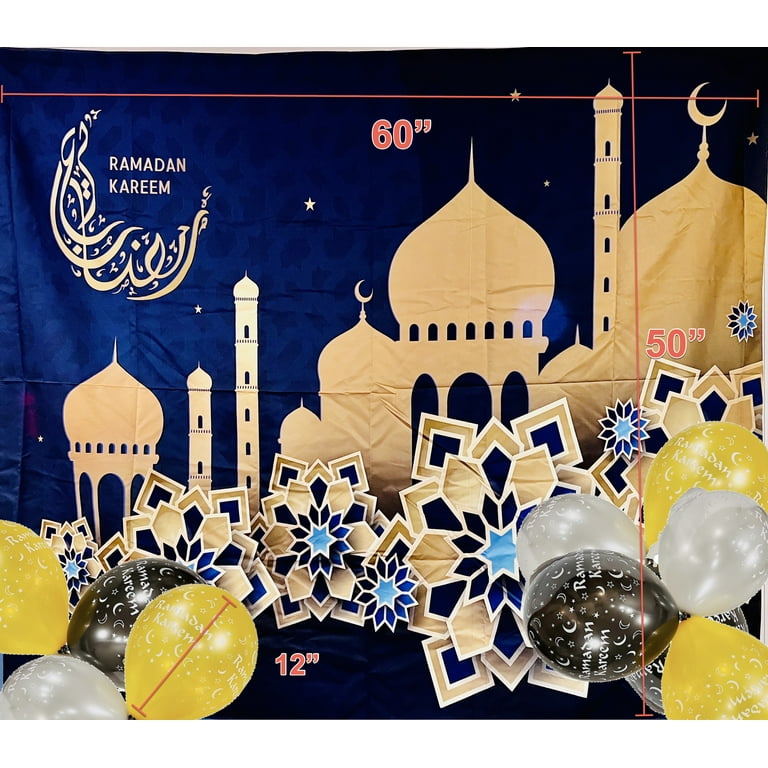This image features a dark blue backdrop or poster adorned with gold silhouettes of mosque-like structures featuring dome-shaped roofs and pointy tips, creating an impression of Middle Eastern architecture. The poster is marked with dimensions: a horizontal line at the top labeled "60 inches" and a vertical line from top to bottom labeled "50 inches," both in an orange font. In the top left corner, the text "Ramadan Kareem" is prominently displayed in light beige, all in capital letters. The backdrop is decorated with snowflake-like patterns in tan and is accompanied by party balloons in yellow, white, and dark brown or black at the bottom.